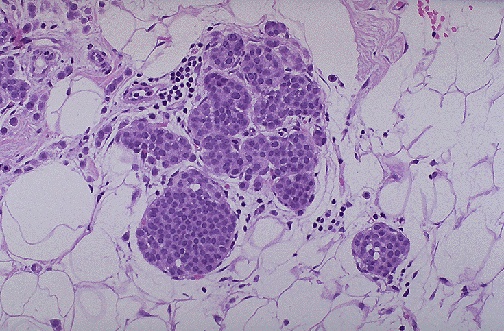This image, seemingly taken under a microscope, displays a close-up of cellular structures that have been stained for better visualization. Predominantly deep purple to dark pink, these irregularly shaped cells are interspersed with darker purple dots within them, indicative of internal components targeted by the dye. Concentrated in the central-left area, a cluster of these cells is surrounded by paler, nearly white circles, creating a stark contrast that highlights the distinct, vibrant purple cells.

Towards the left, these purple cells appear to fragment, with some dark dots spilling out, resembling a river of sorts, possibly hinting at a fluidic movement, perhaps blood. In the broader context of the image, various cells are connected by lighter-hued vessels, forming a network that integrates larger, blob-like structures with interconnected smaller, darker blobs. The overall composition is a mosaic of purples, ranging from deep and intense to light and pale, blending into a visually intriguing yet complex array of cellular forms and connections.